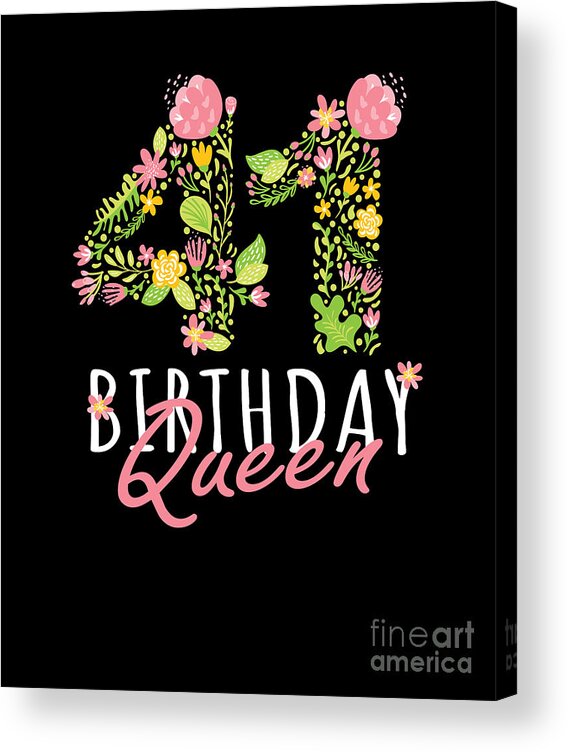The image features a striking black background that highlights the text "41 Birthday Queen." The number "41" is creatively composed of pink, yellow, and orange flowers along with green leaves, adding a natural, colorful touch. These floral elements extend slightly beyond the digits, drawing attention to their intricate design. Surrounding the letters "B" and "Y" in the word "Birthday," small pink flowers are delicately placed, adding to the overall aesthetic. The phrase "Birthday Queen" uses bold, bright pink letters, while "Queen" is depicted in a gold bubblegum color. There is also a soft shadow behind these words, enhancing their visual prominence. At the bottom of the image, the text "Fine Art America" appears in a light gray color, subtly blending with the black background.